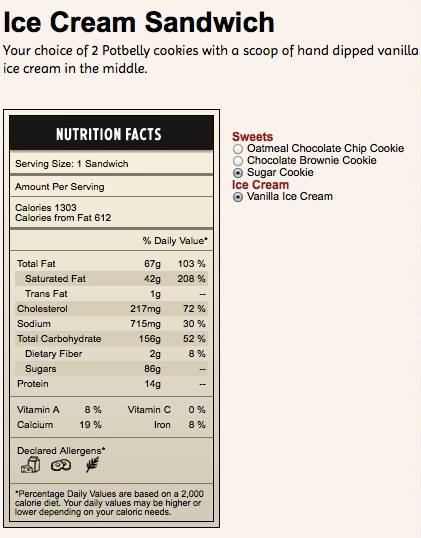This rectangular portrait image features the back of a nutrition panel from a website, showcasing an ice cream sandwich. The background is a light off-white color. At the top left, bold black text reads "Ice Cream Sandwich," followed by smaller left-justified text stating, "your choice of two Potbelly cookies with a scoop of hand-dipped vanilla ice cream in the middle." 

To the lower left, a detailed nutrition facts panel covers about 75% of the height and 45% of the width of the image. It has a black border on top with white text saying "Nutrition Facts." The rest of the panel is a light yellow-brown color with alternating gray lines defining each section. All text within the panel is black. It lists:

- Serving Size: 1 sandwich
- Calories: 1303, with 612 calories from fat
- Total Fat: 67g (103% DV), Saturated Fat: 42g (208% DV), Trans Fat: 1g
- Cholesterol: 217mg (72% DV)
- Sodium: 715mg (30% DV)
- Total Carbohydrate: 156g (52% DV), Dietary Fiber: 2g (8% DV), Sugars: 86g
- Protein: 14g
- Vitamin A: 8%, Calcium: 19%, Vitamin C: 0%, Iron: 8%

Beneath the vitamins and minerals section, the panel indicates declared allergens with small images for milk, eggs, and an unidentified leaf symbol. 

To the right of the nutrition facts, in red text, the word "Sweets" is followed by options including oatmeal chocolate chip cookie, chocolate brownie cookie, and sugar cookie, with the sugar cookie option checked. Below, Ice Cream is also listed in red, with "Vanilla Ice Cream" checked beneath it.